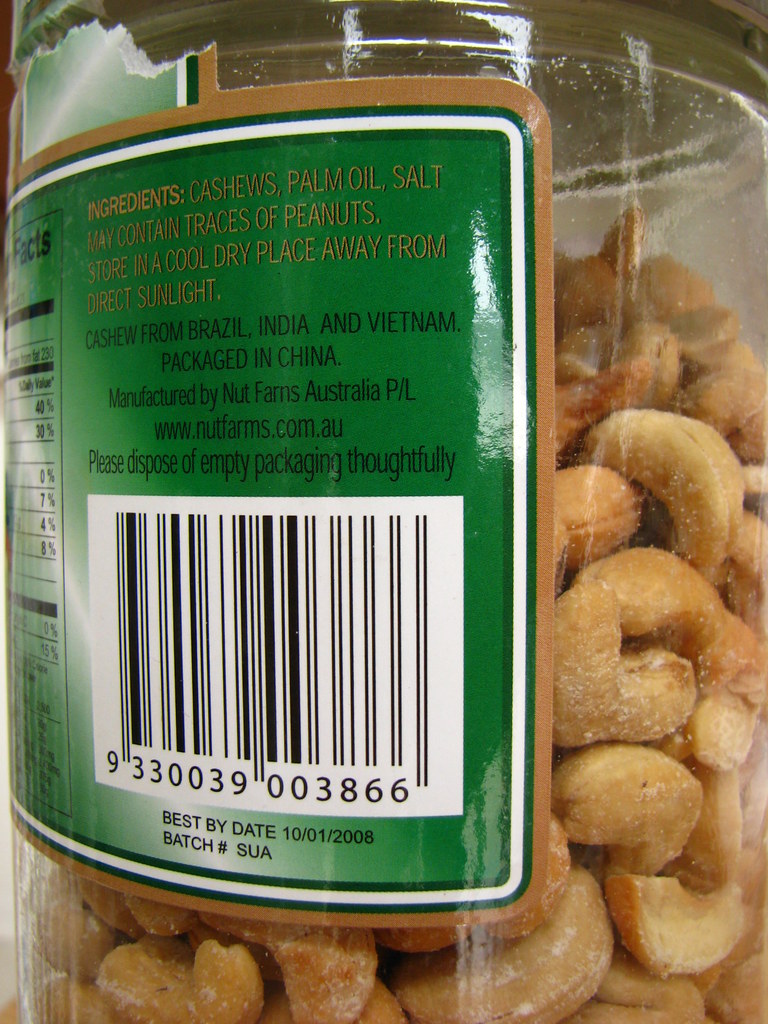This close-up image reveals a jar filled three-quarters with light brown cashews. The clear container prominently displays a detailed label. The label is bordered with a brown trim and features a sequence of stripes - a green stripe followed by a white stripe. The central part of the label is green and lists the ingredients in gold print: "cashews, palm oil, salt. May contain traces of peanuts. Store in a cool, dry place away from direct sunlight". Additional text in black print reads: "Cashews from Brazil, India, and Vietnam. Packaged in China. Manufactured by Nut Farms, Australia, P/L. www.nutfarms.com.au. Please dispose of empty packaging thoughtfully." The label also includes a barcode and notes the "Best by date: 01/10/2008" along with the batch number "SUA." Visible on the left side is a small, partially obscured section of the nutritional facts, though the details are not discernible.